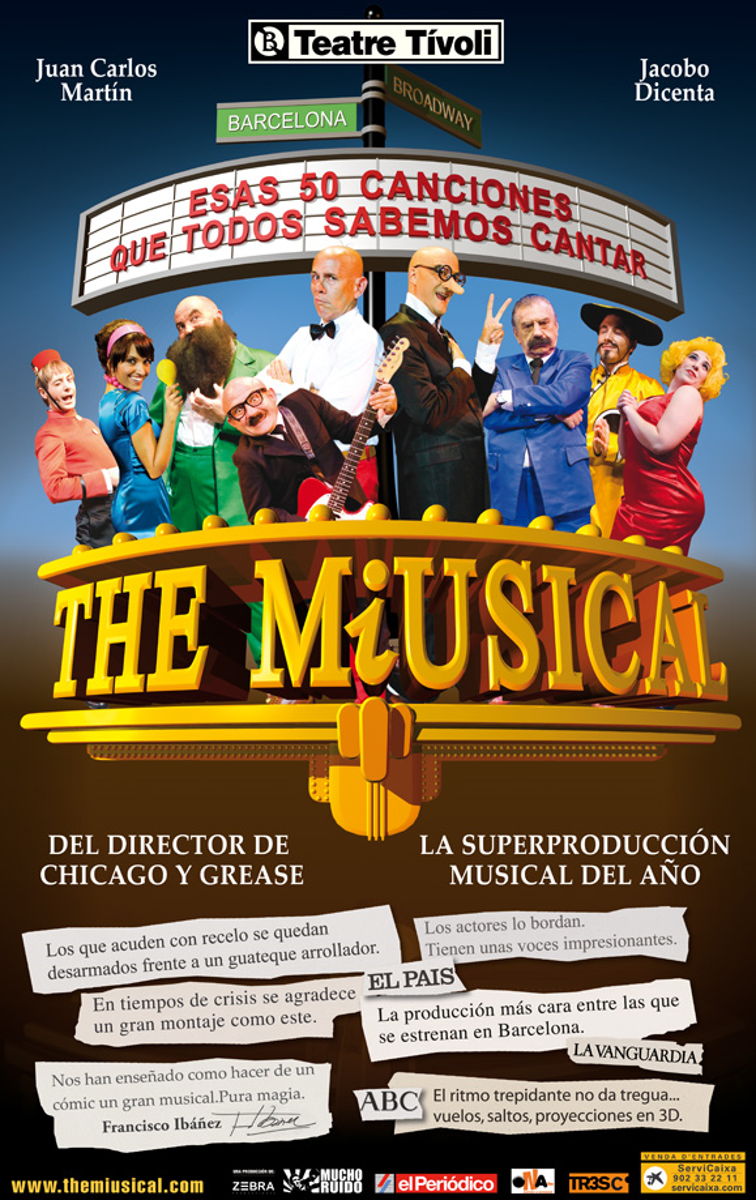This vibrant image serves as an advertisement for a theatrical musical titled "The Musical." It features a large group of men and women, elegantly dressed in suits, tuxedos, and formal dresses, with one man notably playing a guitar. A prominent banner across the top cites both Barcelona and Broadway, suggesting an international flair or crossover production. The text throughout the poster is primarily in Spanish, including information about the Theatre Tivoli, where the musical is being staged. The scene encompasses various characters, including a woman in a striking red dress and a man wearing a sombrero, alongside others in formal attire and even a bellhop. Beneath the central image, the words "The Musical" are prominently displayed, followed by the director's name, indications of critical acclaim through positive reviews, and several company logos at the bottom. Additionally, a website is provided for those interested in more details. The overall design exudes excitement and sophistication, clearly aiming to entice potential theatergoers.